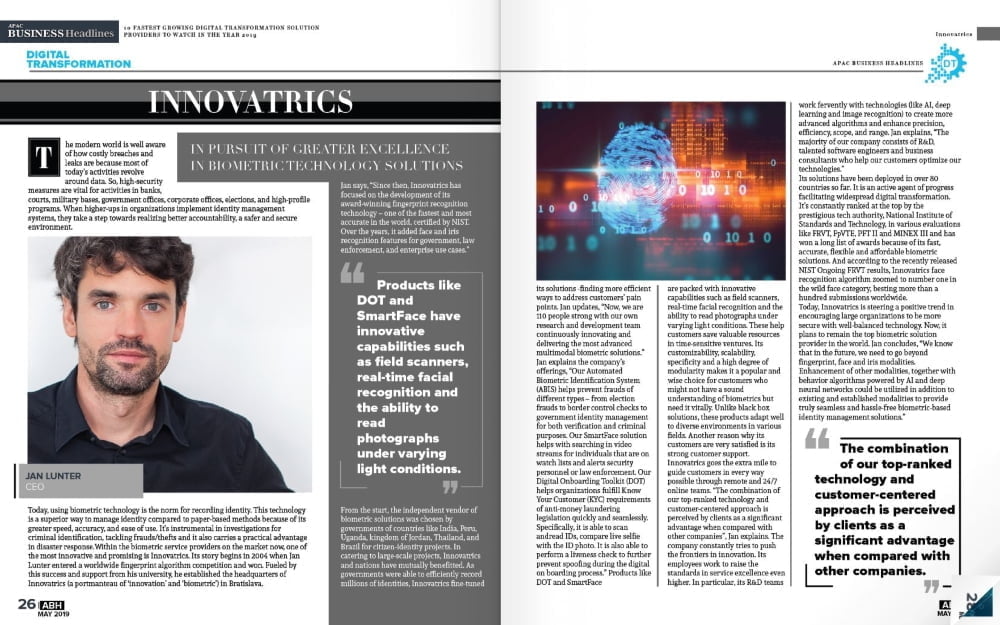This screenshot presents a detailed digital form of a newspaper article, featured in the "Business Headlines" section under the subcategory "Digital Transformation Innovatrix." The article occupies two full pages, densely packed with text that is too small to decipher in the screenshot. However, several prominently enlarged quotes offer key insights into the article's focus. 

One featured quote reads: "Products like Dot and Smartface have innovative capabilities such as field scanners, real-time facial recognition, and the ability to read photographs under varying light conditions." This quote is underscored by the headline, "In pursuit of greater excellence in biometric technology solutions."

Accompanying the article are a couple of photographs. On the left side of the first page, a photo of a male figure is labeled "Jan Lunter, CEO." The second page includes an image on the right, depicting a fingerprint overlaid with digital numerals of ones and zeros, symbolizing biometric technology.

Overall, the article delves into the advancements and potential of biometric technologies through the innovative products Dot and Smartface, as articulated by industry leader Jan Lunter.